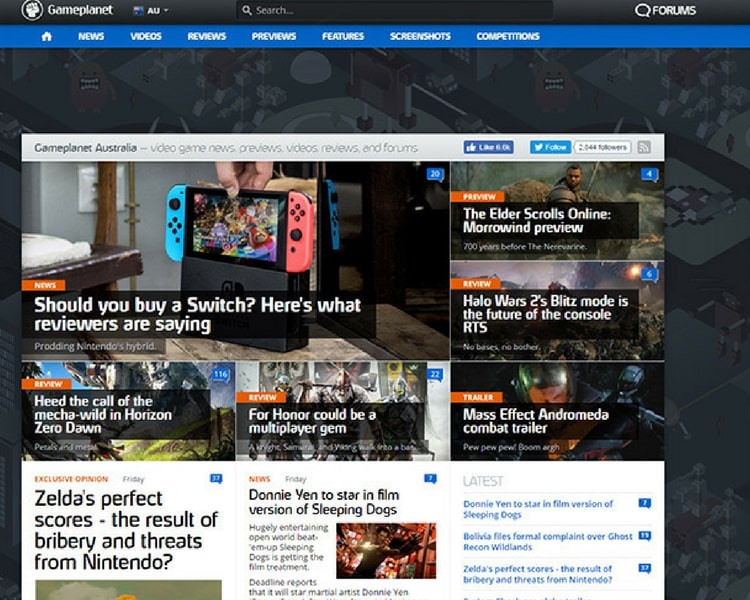This image showcases the homepage of a website named "Game Planet Australia." The header prominently displays the logo and tagline: "Game Planet Australia - Video Game News, Previews, Videos, Reviews, and Forums." In the top area, there is a search bar, a section for forums, and navigational options.

Highlighting the main content, the top article poses the question, "Should you buy a Switch? Here's what reviewers are saying." Adjacent to this on the upper right side, there's a preview titled "The Elder Scrolls Online: Morrowind Preview." Below, another article catches attention with the headline, "Halo Wars 2's Blitz Mode: The Future of Console RTS's."

Descending to the left side of the page, an article reads, "Heed the Call of the Mecha Wild in Horizon Zero Dawn." Shifting focus to the central part, "For Honor Could Be a Multiplayer Gem" is featured prominently. Over to the far right, the headline "Mass Effect Andromeda Combat Trailer" invites readers to explore further.

At the bottom of the page, three additional sections offer a variety of articles for in-depth reading, rounding out the diverse content available on the homepage.